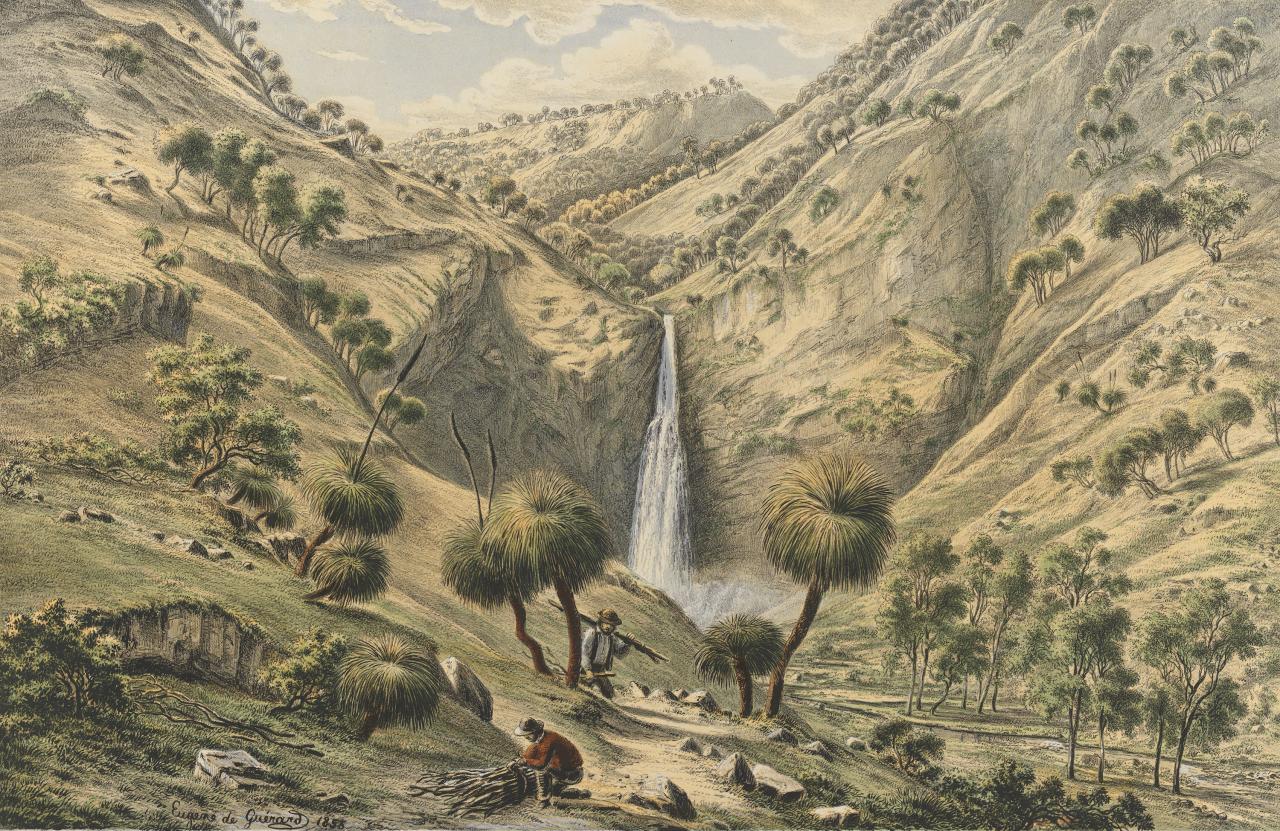This detailed painting by Eugene von Guerard, titled "Fall of the First Creek" near Glen Osmond in South Australia, captures an exquisite and lush natural scene. Dominating the image is a steep, verdant valley flanked by hillsides brimming with Australian-looking trees. In the very center of the painting, a tall, narrow waterfall cascades down between these forested slopes. The water lands into a barely visible pool, adding to the serenity of the landscape. The sky above is a mix of blue and white clouds, presenting a slightly desaturated hue that complements the overall light green tone of the terrain.

In the foreground, amid a rocky patch, two men are engaged in what appears to be harvesting or gathering wood. One man, donned in a red and white shirt with long sleeves and a hat, carries a large forked stick, while the other, also in long sleeves and a hat, is crouched, tying up some wood on the ground. Their faces remain indistinct. This serene, yet industrious scene is devoid of any textual descriptions, allowing viewers to fully immerse themselves in the natural beauty and human activity depicted.